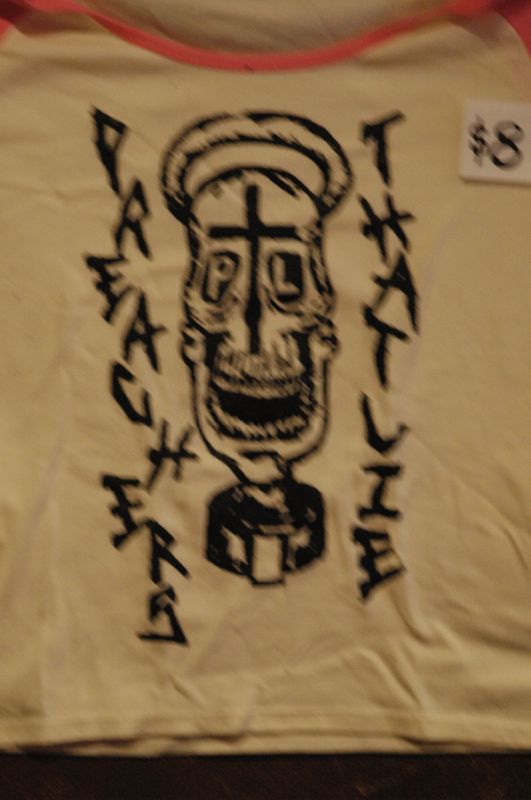This photograph captures a wrinkled white t-shirt laid flat on a surface, viewed from above in a blurry, out-of-focus manner. The shirt features a prominent pink border around the collar and pink sleeves, with the pink areas visible at the shoulders and the very top edges of the sleeves. 

A small white square price tag positioned on the bottom right shoulder prominently displays the cost of "$8" in large, black font, nearly filling the entire tag.

The centerpiece of the shirt is an extensive graphic that spans from just below the neckline down towards the bottom. This graphic depicts a long, narrow skeleton face adorned with a chef's hat. The skeleton's face is marked by a large vertical cross running from its forehead, over the nose, and down to the top lip, with a horizontal line intersecting above the eyebrows, giving the appearance of a unique expression. Below the face, the skeleton's mouth, filled with numerous teeth, forms a characteristic smile. It sits on a circular base designed to resemble a trophy. 

Surrounding the skeleton graphic, intense "punk rock" styled letters spell out "PREACHERS" vertically on the left side and "THAT LIE" vertically on the right side. The shirt exhibits visible wrinkles towards the bottom right and left sections, adding texture to the overall appearance.